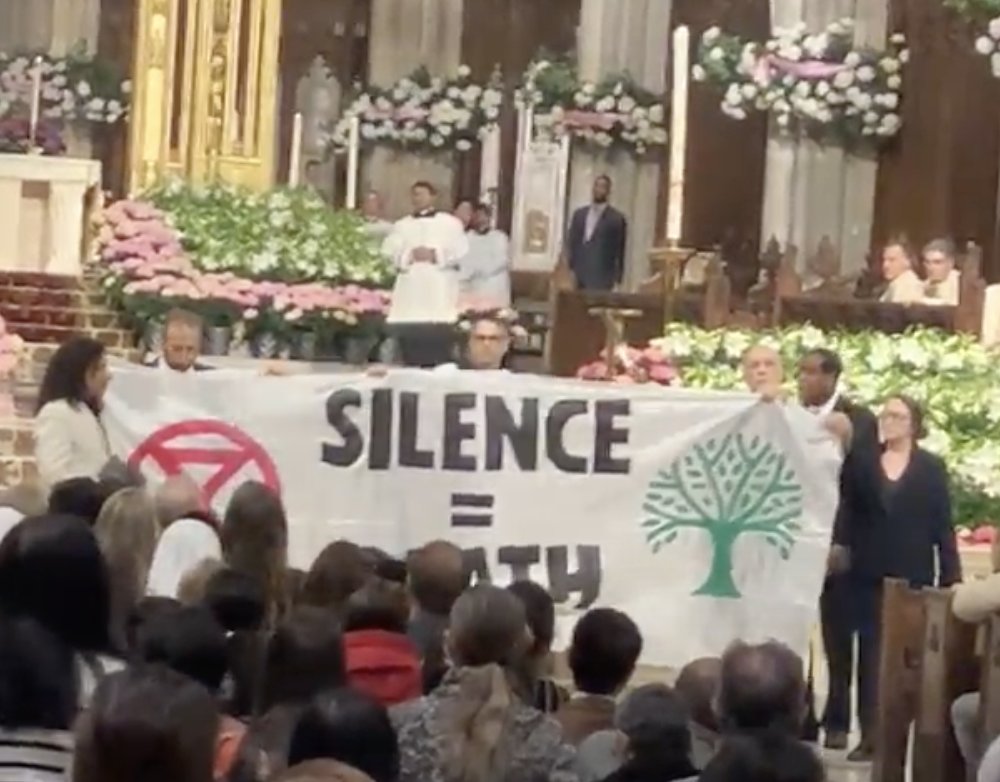The image captures the inside of a church during a significant event. At the forefront, a diverse group of people holds up a large banner partially obscured by the heads of seated audience members. The banner reads "Silence equals TH," likely "death," and features a green clip-art tree on its right side. Adjacent to the tree is a red circle with a red triangle inside. The individuals holding the banner include a woman with her hair up, dressed in a black suit and glasses, and another woman in a white blazer with long brown hair. Behind them, numerous bouquets of flowers with pink ribbons and green leaves adorn the stage and altars, adding to the scenery of the ceremony. A minister in a white robe stands prominently on the stage, framed by lit candles, and possibly joined by other clerical figures in white gowns with dark collars. Further back, more participants, possibly choir members or congregants, are seated at a higher elevation. The attentive audience, viewed from behind, fills the lower part of the image, creating a full and detailed depiction of this church gathering.